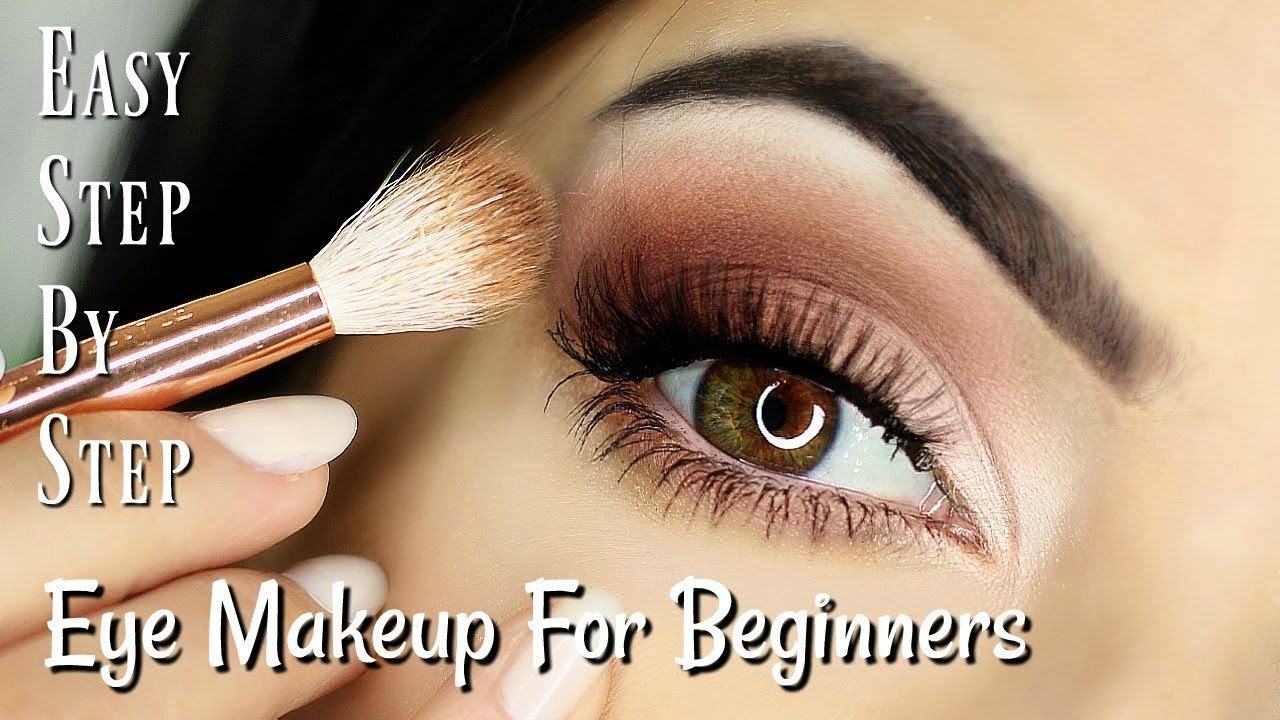This image is a close-up shot forming the thumbnail for a YouTube or TikTok video, aimed at beginners seeking to learn eye makeup application. The text on the thumbnail, "Easy Step-by-Step" written vertically on the top left, and "Eye Makeup for Beginners" written horizontally at the bottom, clearly indicates the instructional nature of the content. The woman's eye, a captivating mix of brown and hazel with hints of green, is the focal point. She has long, beautiful eyelashes and meticulously manicured eyebrows and nails, with the nails painted white. The makeup being applied is a blend of bronze and lighter shades, expertly blended to show a gradient from flesh color to darker brown. In the reflection of her eye, a ring light is visible, suggesting a professional setup likely for video content creation. Her brown hair is partially visible, completing the aesthetic of a well-curated beauty tutorial.